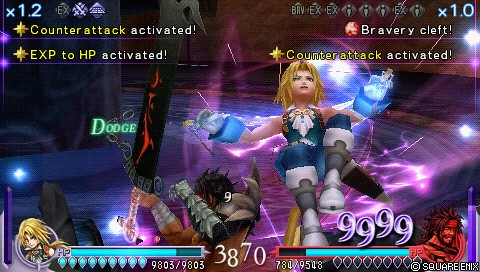This is a detailed screen capture from a video game, prominently displaying the "Copyright Square Enix" watermark in the lower right-hand corner. The upper portion of the screen is adorned with several important text overlays in white, including "Counter Attack Activated," "EXP to HP Activated," "Bravery Cleft," and another "Counter Attack Activated." 

The central focus of the image is a female character. She sports blue wristbands and a distinctive white glove, which appears to emit a faint glow, particularly on her left hand. Her pose is dynamic, with her left leg raised and bent at the knee, suggesting she is mid-action. Her face, intriguingly, is covered with a mask resembling a dog's face, complete with goggles, adding an element of mystery and fantasy. She is dressed in a sleeveless uniform-style outfit that enhances her agile and combat-ready appearance.

In the lower left corner, another character is visible, enclosed within a circle, possibly indicating a selectable or highlighted ally or enemy. The scene is saturated with vivid images, lights, and a rich palette of purples and blues, contributing to the game's immersive and fantastical environment. The word "Dodge" is prominently displayed, located at the left center of the screen, likely a prompt or indication related to the gameplay mechanics.